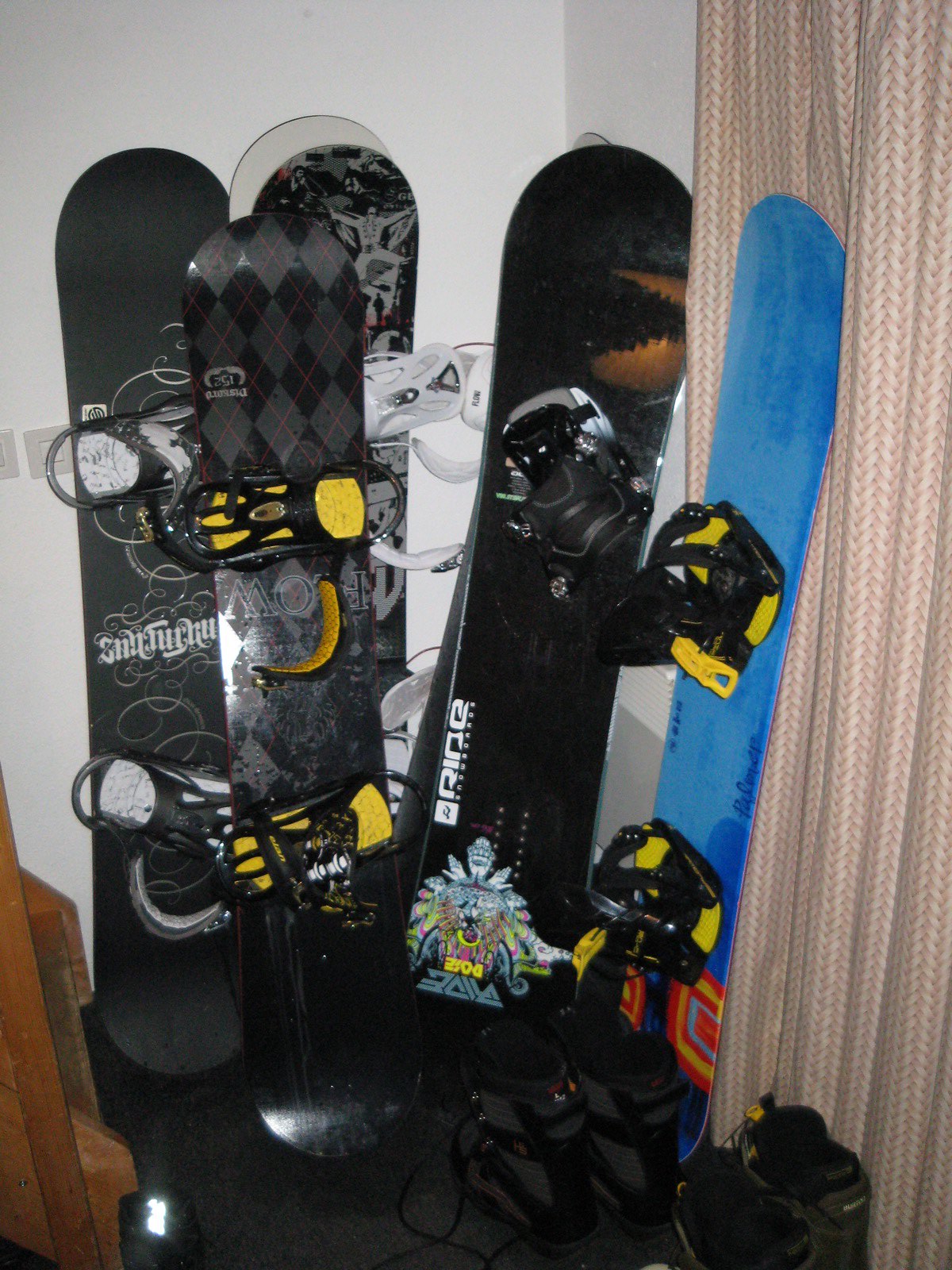This detailed indoor photo features a scene centered around several snowboards propped against a white wall. On the right side, a cream (or brown-and-white) colored curtain hangs down the length of the wall, juxtaposed next to a set of light switches in the middle of the left wall. The light fixtures appear in a grayish hue. The floor, visible at the bottom left of the image, showcases a light brown, wooden texture.

In the foreground, multiple snowboards are prominently displayed. Starting from the left, the first snowboard is black with white text and scribbles. Adjacent to it is another black snowboard, featuring a distinctive diamond-checker pattern in black and gray, and yellow footstraps designed for boots. Next is a snowboard bearing the word "R.I.D.E." in bold white letters. Further to the right, there is a snowboard that showcases a colorful character design with a big yellow belt and silver text on the bottom. A final snowboard leans against the curtain, predominantly blue with orange, yellow, and red accents at the bottom.

In the lower corner of the image near the steps, you can also spot black snow boots, hinting at the snowboarding activity. The overall scene depicts an organized space with a clear emphasis on snowboarding equipment against a backdrop of homey indoor elements.